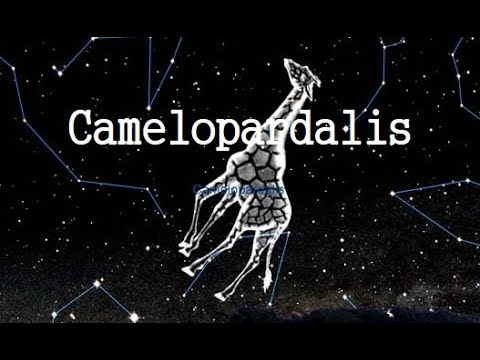The image is a detailed digital illustration, resembling a screen capture or a PowerPoint slide, that artistically depicts the constellation Camelopardalis. The background is a dark, star-studded sky with several unnamed constellations outlined by lines between stars. At the center of the image floats a fully illustrated giraffe, glowing with a white aura. This giraffe leans backward and gazes upward toward the upper center of the composition, angled at about 15 to 20 degrees. The sky is predominantly rendered in black and white with subtle hints of light blue. Overlaying the image, the word "Camelopardalis" appears in white lettering, signifying the Latin name for the giraffe constellation. The giraffe's presence amidst the stars visually emphasizes the constellation's form and placement in the night sky.